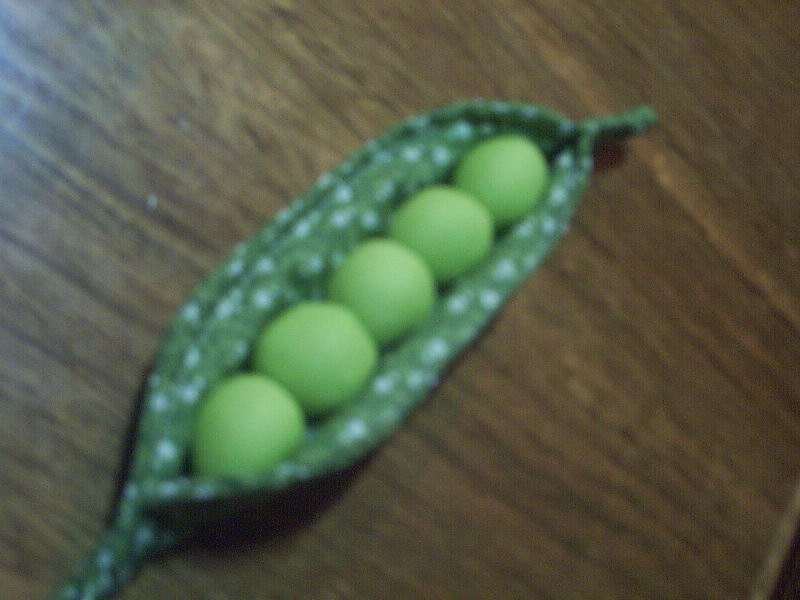This close-up, slightly blurry photograph features an open, green pea pod with white speckles on it, positioned diagonally at the center of the image. Inside the pod, there are five lime green peas that almost resemble small green apples due to their unusual coloration. The texture and appearance of the pod and peas suggest that this might be an arts and crafts item as opposed to a real vegetable. The white speckles and the lime green hue of the peas deviate from the natural look of typical pea pods. The background consists of a brown wooden surface, possibly a table or cutting board, with varying darker and lighter stripes running through it. The image's macro or micro shot perspective contributes to its blurriness and glisten-like appearance.